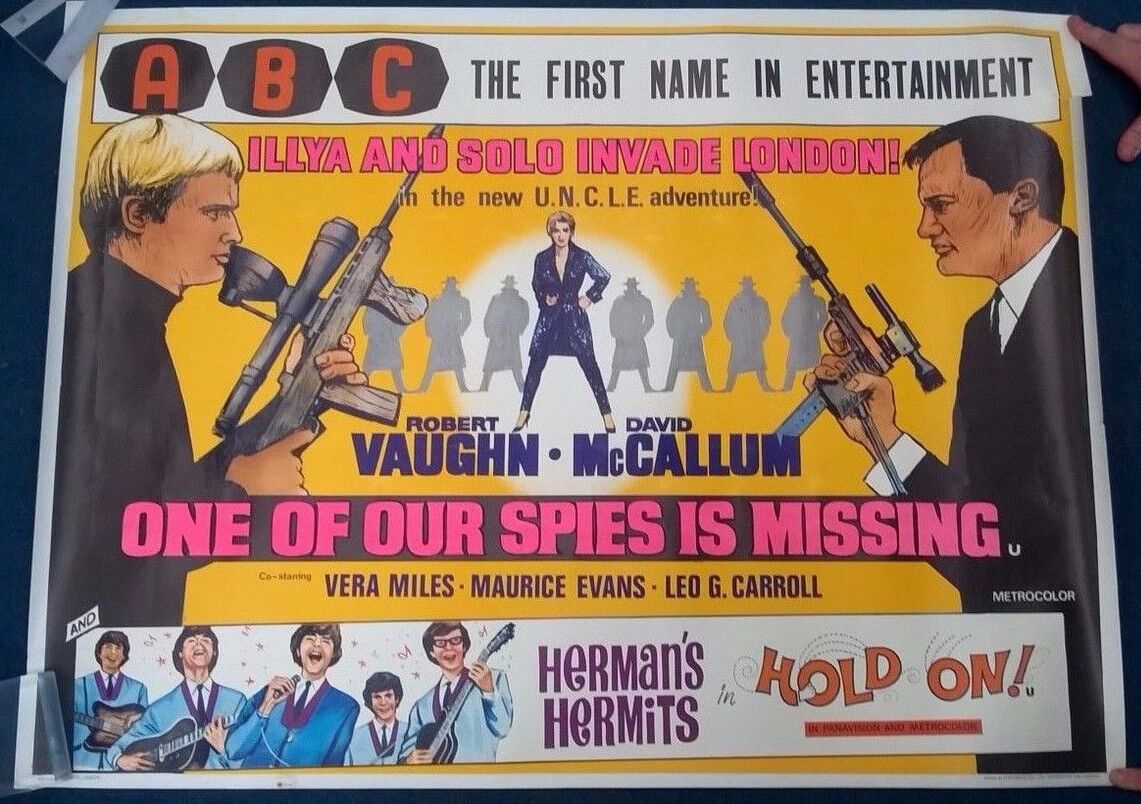This vintage movie poster features a striking hand-drawn design reminiscent of the 1950s-1960s style. The top section has a white banner with the label "ABC" in red, set against black hexagon backgrounds, followed by "The first name in entertainment" in black letters. Below, colorful pink lettering on a yellow background announces, "Ilya and Solo invade London in the new UNCLE adventure!" The central figure is a woman with short dark blonde hair, clad in a black trench coat and leather pants, brandishing a gun, and posed with confidence. Flanking her are two men with automatic weapons: one on the left, blonde and wearing a black turtleneck, and the other on the right, dark-haired and donning a black suit with a white shirt and black tie. Behind them, gray silhouettes of men in trench coats and hats add an air of intrigue. The names "Robert Vaughn" and "David McCollum" are prominently displayed, alongside the intriguing subheader, "One of our spies is missing." At the very bottom, another section showcases band members in blue suits, promoting "Herman's Hermits in Hold On!"